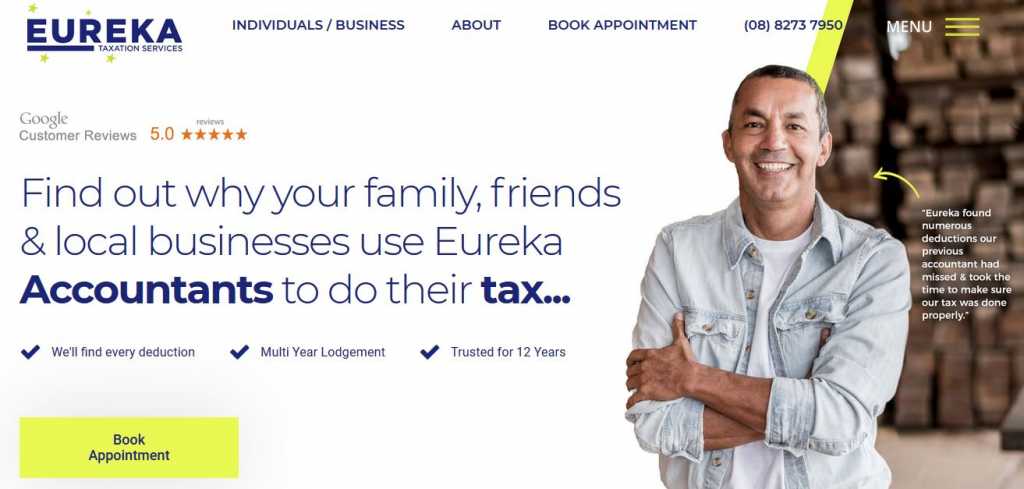This is an image taken from a web page for "Eureka Taxation Services." The company's name is prominently displayed in the top left corner. The navigation bar at the top includes tabs such as "Individuals," "Business," and "About." On the right side of the navigation bar, there is a "Book Appointment" option and the phone number (08) 8273-7950. The upper right corner features a menu button comprising three horizontal yellow bars.

Below the navigation bar, there is a section for Google Customer Reviews with a five-star rating. A navy blue text reads, "Find out why your family, friends, and local businesses use Eureka accountants to do their tax..." with clickable areas that highlight services like "We'll find every deduction," "multi-year lodgement," and being "trusted for 12 years." The bottom lower corner has a yellow "Book Appointment" button in blackish navy print.

The right side of the image features a picture of a man standing with his arms crossed, enhancing the professional yet approachable vibe of the service.